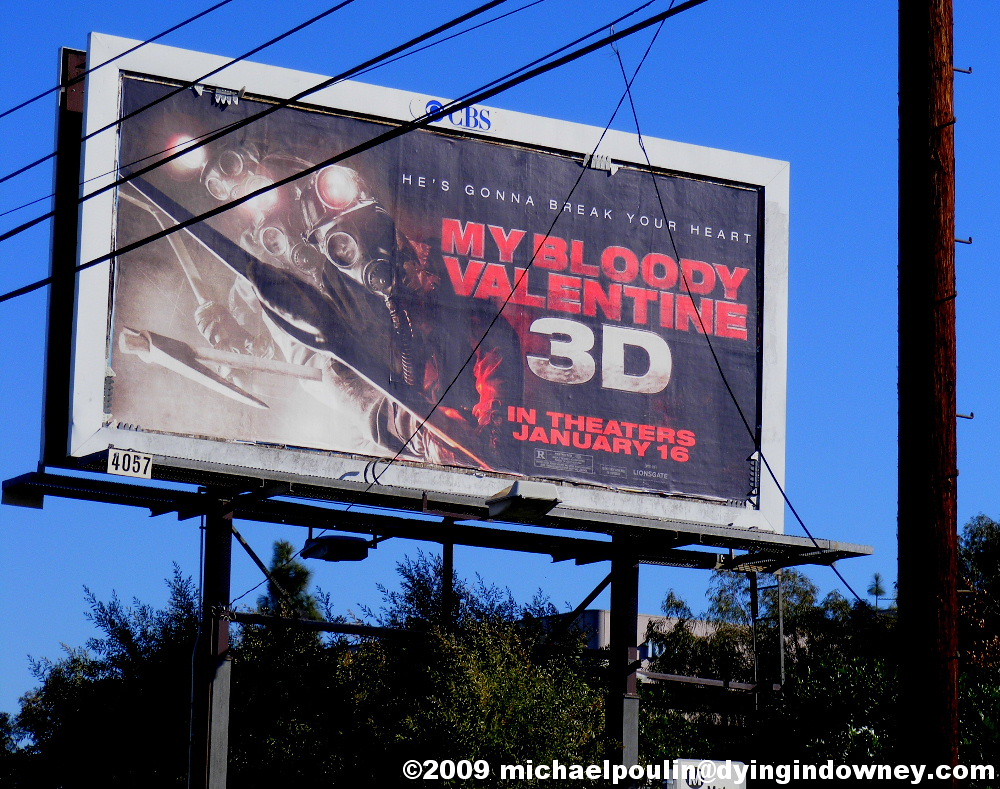The photograph, taken outside during the day, captures a large billboard set against a vividly blue sky. In the upper left-hand corner, four power lines slant diagonally across the image. The billboard is framed in white and exhibits a dark or grayish background at its top section, where the blue letters "CBS" are prominently displayed. Below this, the main graphic of the advertisement features a person wearing a gas mask with a light on top, holding what appears to be a weapon, likely a sword. The right side of the billboard features the text "He's Gonna Break Your Heart" in white, with "My Bloody Valentine" in red beneath it, followed by "3D" in white. The bottom of the billboard announces "In Theaters January 16" in red letters. Additional smaller text at the bottom, which includes "2009 Michael Poland" and a web address "dying in Downey calm," can also be noted. The scene is completed with tree tops visible below the sign, lending a suburban context to the image.